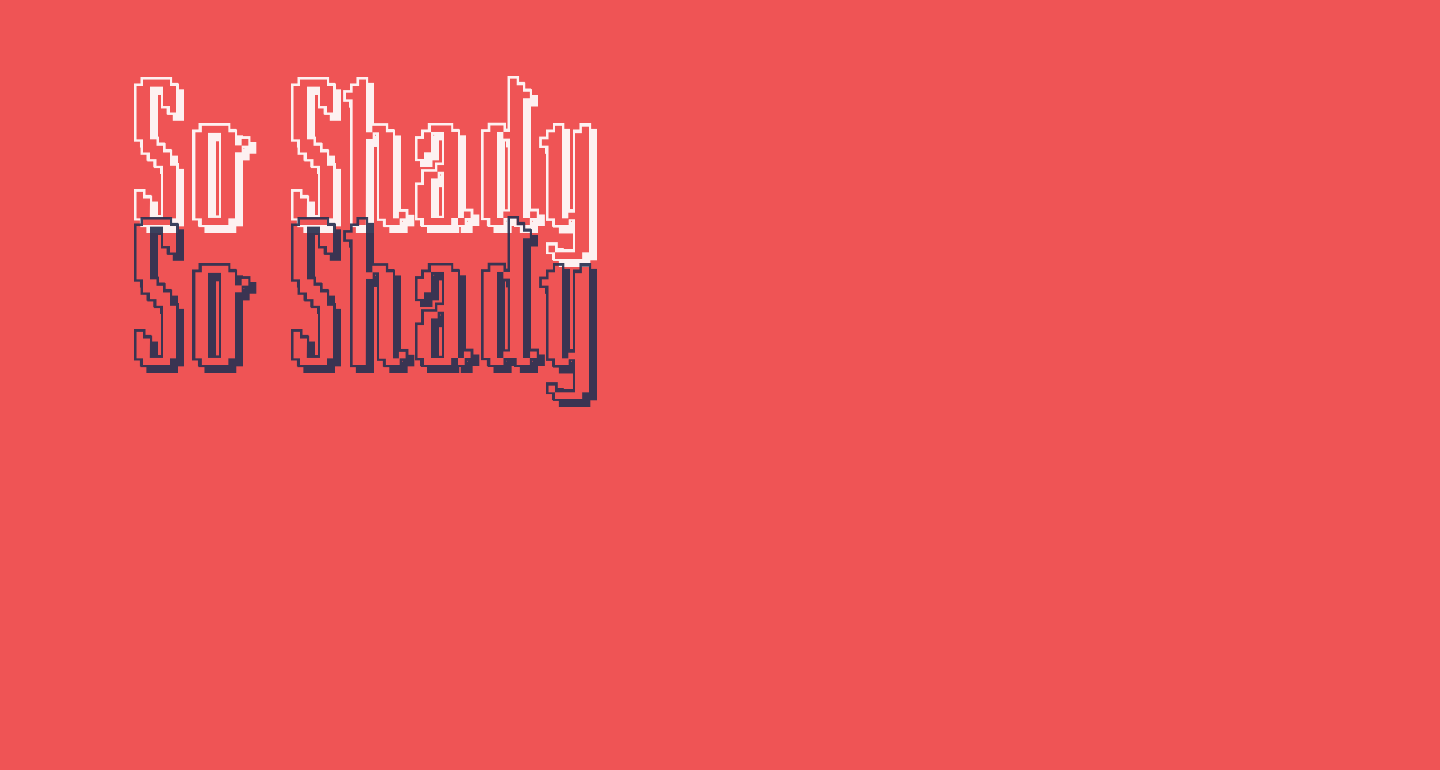The image is a long rectangular graphic with a solid background in a deep coral or blood orange color, giving it a vibrant, warm appearance. In the top left corner, occupying roughly a quarter of the space, there is text repeated twice with a slight overlap. The top iteration of the text reads "So Shady" in outlined white lettering, with hollow centers. Directly beneath and barely overlapping is the same phrase, "So Shady," this time in a dark navy blue. The rest of the image is devoid of any other elements or designs, focusing solely on the contrasting text, hinting at a minimalist aesthetic.